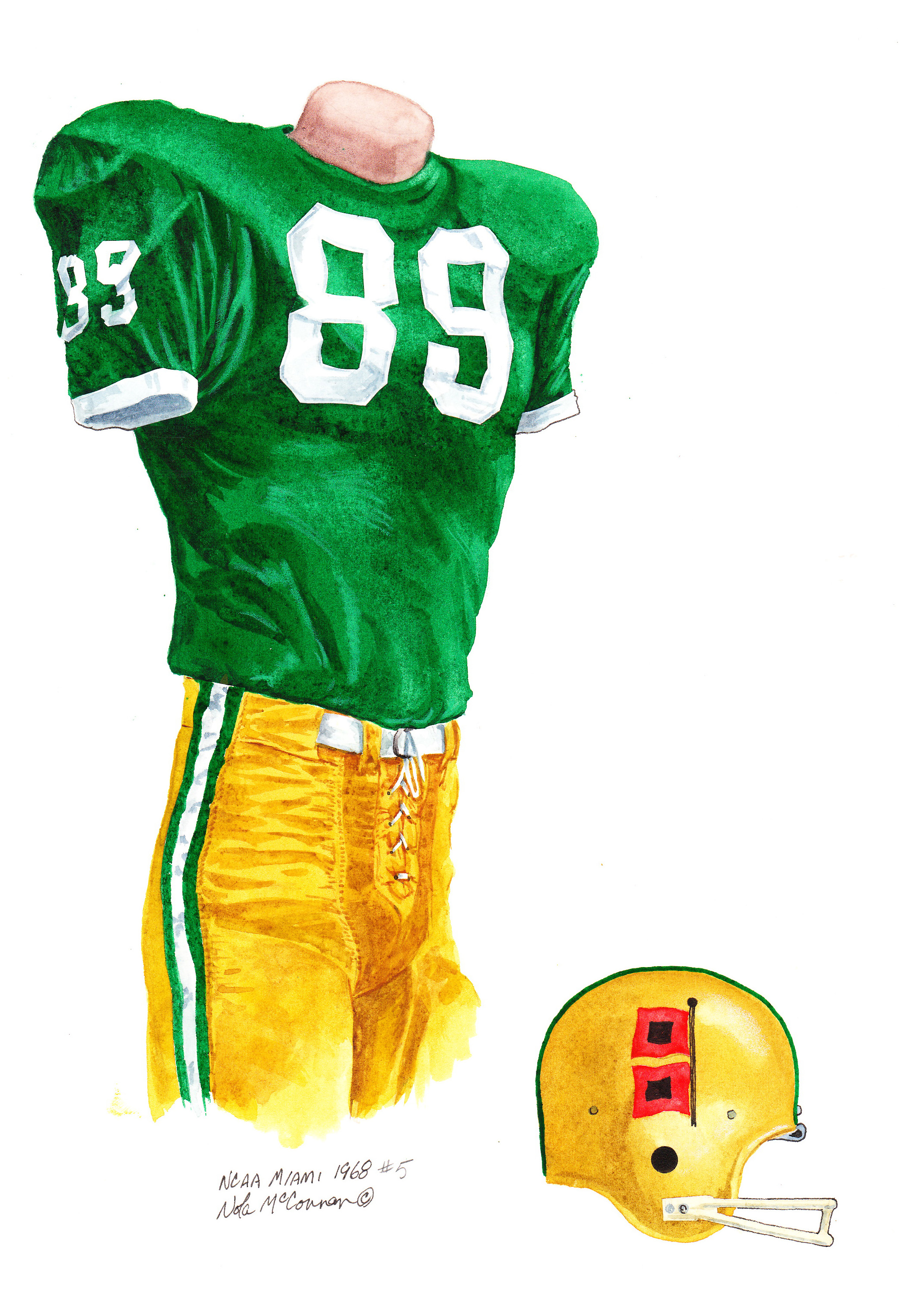The image is a detailed painting or illustration of a headless mannequin dressed in a vintage football uniform. The jersey is a vibrant green with a prominent white "89" displayed on the front and on the right sleeve. The pants are gold, featuring a distinctive white lace-up fly area, accompanied by a white belt and a white-and-green stripe running down the side of each leg. Adjacent to the mannequin is a gold helmet, marked with a green stripe running from the front to the back at the top. Notably, a black pole with two red flags, each featuring a central black square, is also part of the composition. The background is a plain white, allowing the elements of the artwork to stand out. In the lower left-hand corner of the image, the text reads "NCAA Miami 1968 number 5," with the name "Nate McCannon" faintly recognizable. The piece encompasses a range of colors including white, green, gold, red, and black, suggesting it has been meticulously painted by hand.